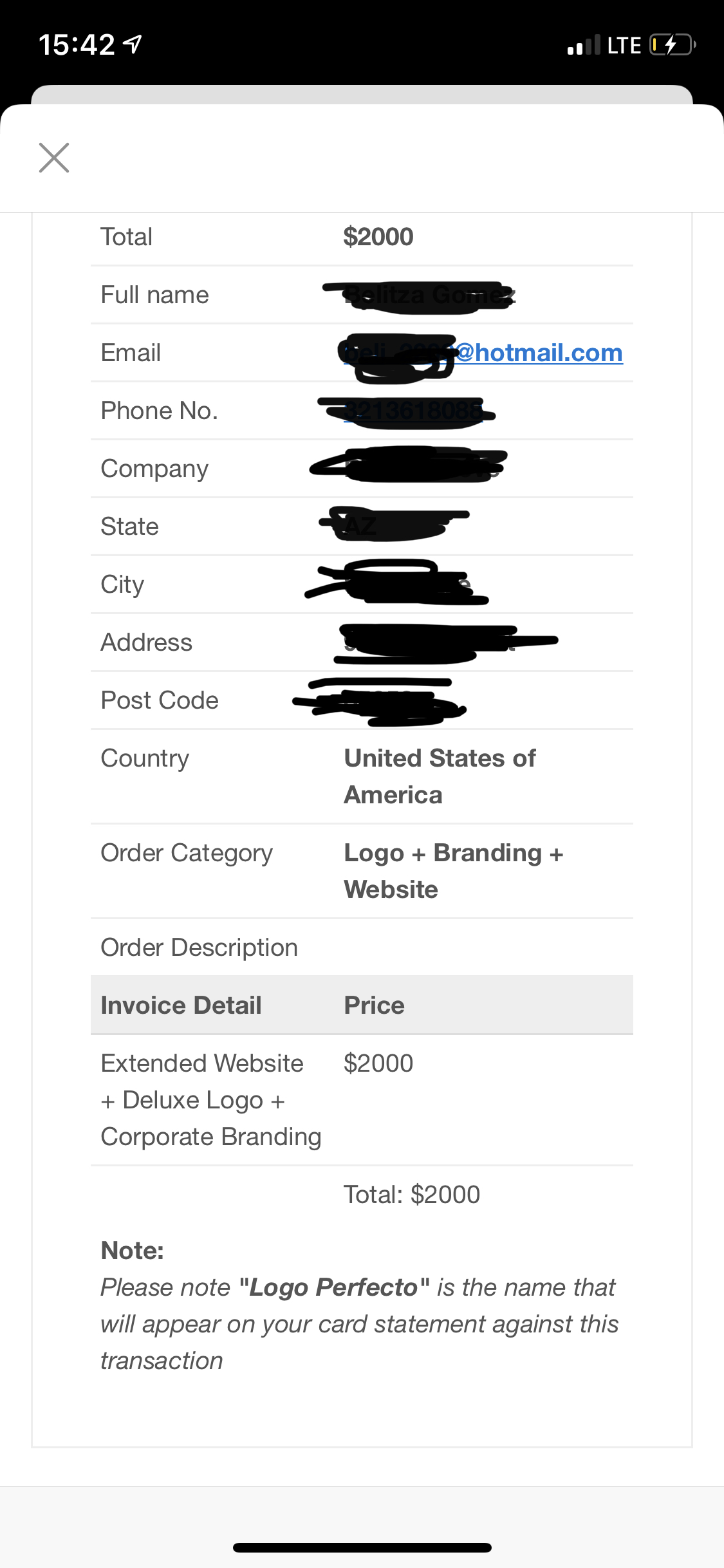The image appears to be a screenshot from a phone, capturing an invoice or order summary. At the very top, the status bar displays various indicators: the time reads "15:40:42" in military format, there's an upward-angled arrow icon, two signal bars accompanied by "LTE" indicating the network status, and a battery icon showing it's charging with a lightning bolt symbol.

Below the status bar is a thin-bordered white rectangle containing detailed invoice information. The total amount due is listed as $2,000. The subsequent fields, which are all partially redacted, likely include the customer's full name, email (ending in "@hotmail.com"), phone number, company, state, city, address, postcode, and country (listed as "United States of America").

Further down, the order details specify the category as "logo, branding, and website." The invoice details are segmented by alternating white and gray backgrounds. The first entry on a gray background includes "invoice detail, spaces, price," followed by the specifics on a white background: "Extended website: $2,000" and "Deluxe logo + corporate branding." The total amount reiterated is $2,000.

A note at the end of the invoice, enclosed in quotation marks, states: "Please note, 'Logo Perfecto' is the name that will appear on your card statement against this transaction." Finally, a black bar runs horizontally across the bottom of the image.